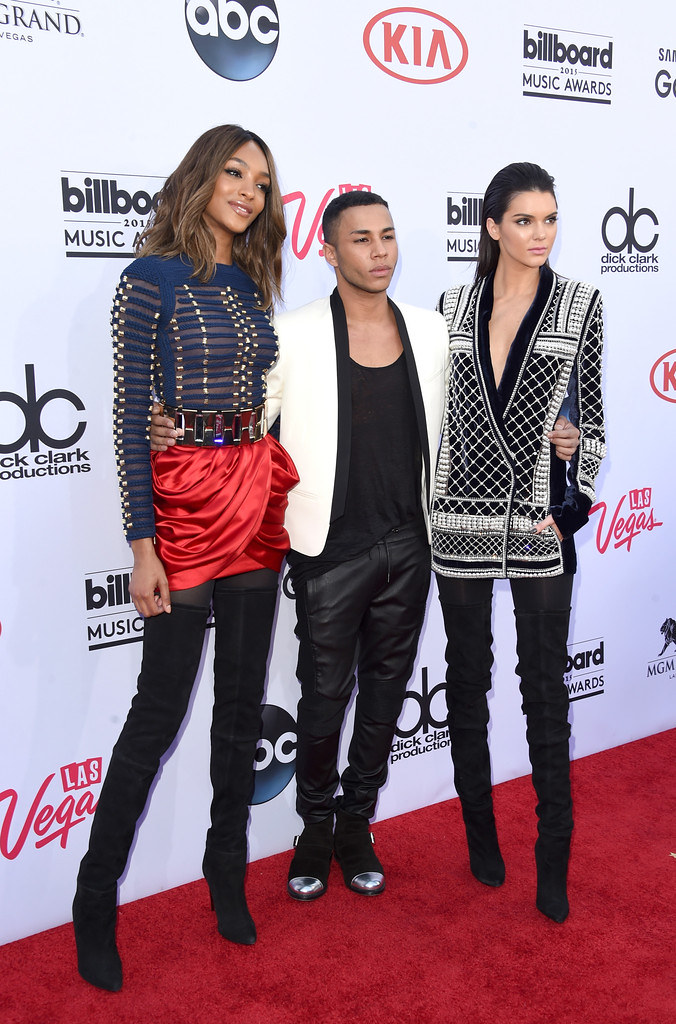In this red carpet photograph taken at the Billboard Music Awards, a striking trio poses confidently in front of a white backdrop adorned with logos such as ABC, Kia, Las Vegas, and Dick Clark Productions. At the center is a short, brown-skinned young man sporting black leather pants, a black t-shirt, and a distinctive white blazer. On his right, Kendall Jenner stands out with her black hair pulled back, dressed casually in a black and white loose-fitting top, black skinny jeans, and tall black boots. To his left is a tall, model-esque black woman wearing a blue top with gold buttons, a shiny red skirt, and thigh-high black boots. Behind them, the branded backdrop repeats its logos in a sleek tiled pattern, setting the stage for this glamorous event.